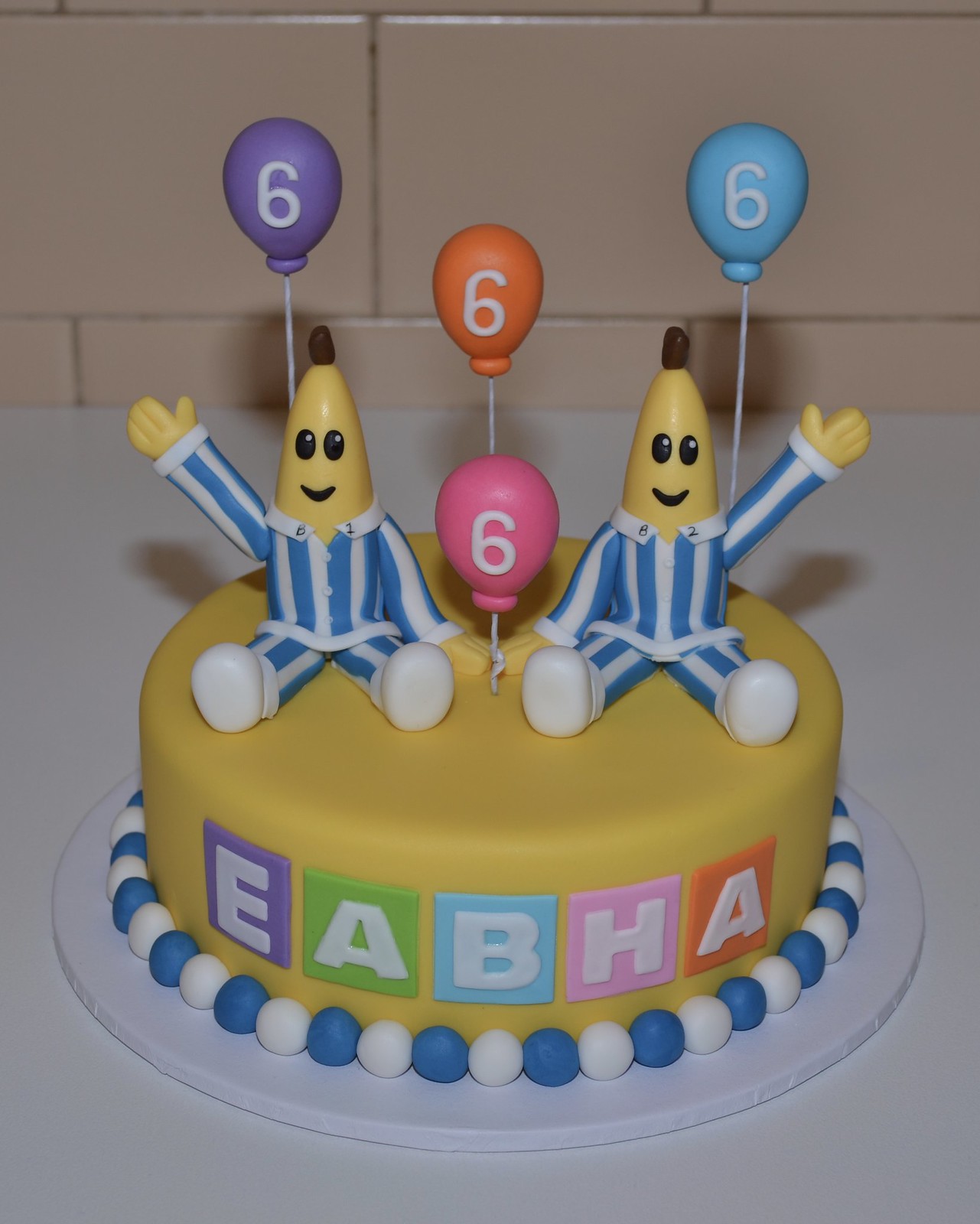This color photograph showcases an elaborate children's birthday cake prominently featuring characters from the classic "Bananas in Pajamas" cartoon series. The single-layer cake is covered in smooth, yellow fondant icing, adorned with blue and white fondant beads around its base. The front of the cake displays the letters "E-A-B-H-A," each letter set within a uniquely colored block. Topping the cake are two identical "Bananas in Pajamas" figurines, dressed in blue and white striped pajamas with white shoes. These figurines are seated, each extending one arm outward. The figures have brown tufts on top of their heads and friendly facial expressions. Also on top of the cake are four colorful balloons—purple, orange, pink, and blue—each inscribed with the number six, indicating the age being celebrated. The cake rests on a white countertop against a backdrop of tan or light pink tiles, adding a homey touch to the celebratory scene.